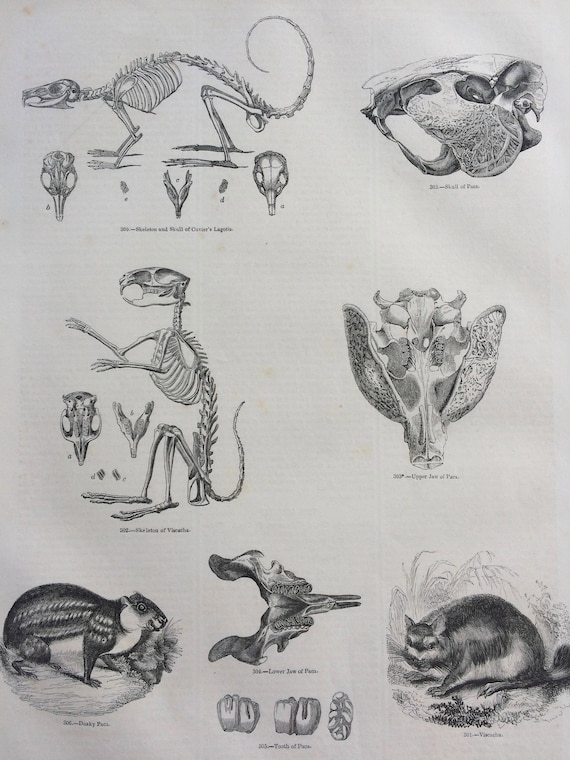The detailed image displays seven monochrome pencil illustrations on a light gray background, focusing on the anatomy of a rodent-like animal, possibly a squirrel or gopher. In the top left corner, the full skeleton of the creature is depicted from a side view, facing left. To the right of this, the skull of the animal is illustrated, also facing left. In the bottom right corner, the live creature is shown in a natural outdoor setting. The bottom left corner features the same creature, now facing right. Above this, there's another full-body skeleton of the creature, appearing to sit on its hind legs with both arms raised. Each drawing is detailed and professional, akin to what might be seen in an animal or art museum, with black text labels beneath each illustration explaining the different views and parts of the animal’s anatomy.